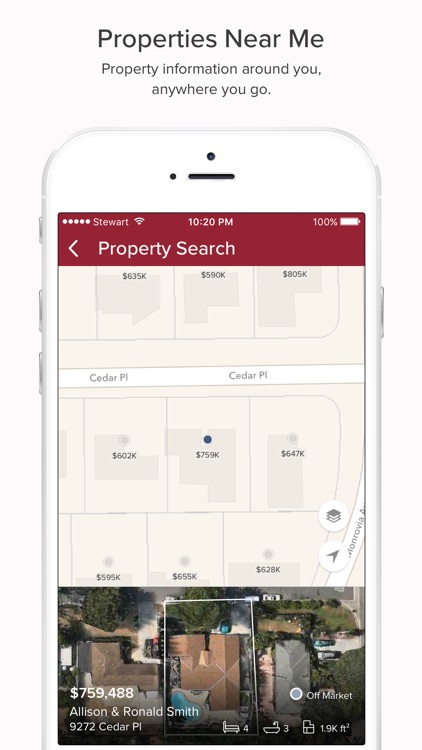The image is a vertically-oriented photograph featuring a white smartphone against a lighter gray background. The phone's display showcases an app with property listings, titled "Properties Near Me: Property Information Around You, Anywhere You Go," prominently displayed at the top. The phone, slightly truncated at the bottom, reveals the volume and power buttons on the side.

On the screen, the status bar at the top includes essential icons: signal bars and a Wi-Fi icon on the upper left, the time "10:20 PM" in the center, and a fully charged battery icon on the upper right.

Below the status bar, a red rectangle highlights a property search interface. The search results feature multiple property listings with prices such as $635,000, $590,000, and $805,000, accompanied by street addresses. Each listing is marked with small blue dots, indicating more properties such as $602,000 and $795,000. One specific listing stands out with a price of $647,000 and another, which appears highlighted, shows $759,488 along with its address and a small thumbnail image.

The detailed display and clear layout of the phone screen provide a comprehensive overview of available properties, making it easy for users to navigate and explore potential homes.